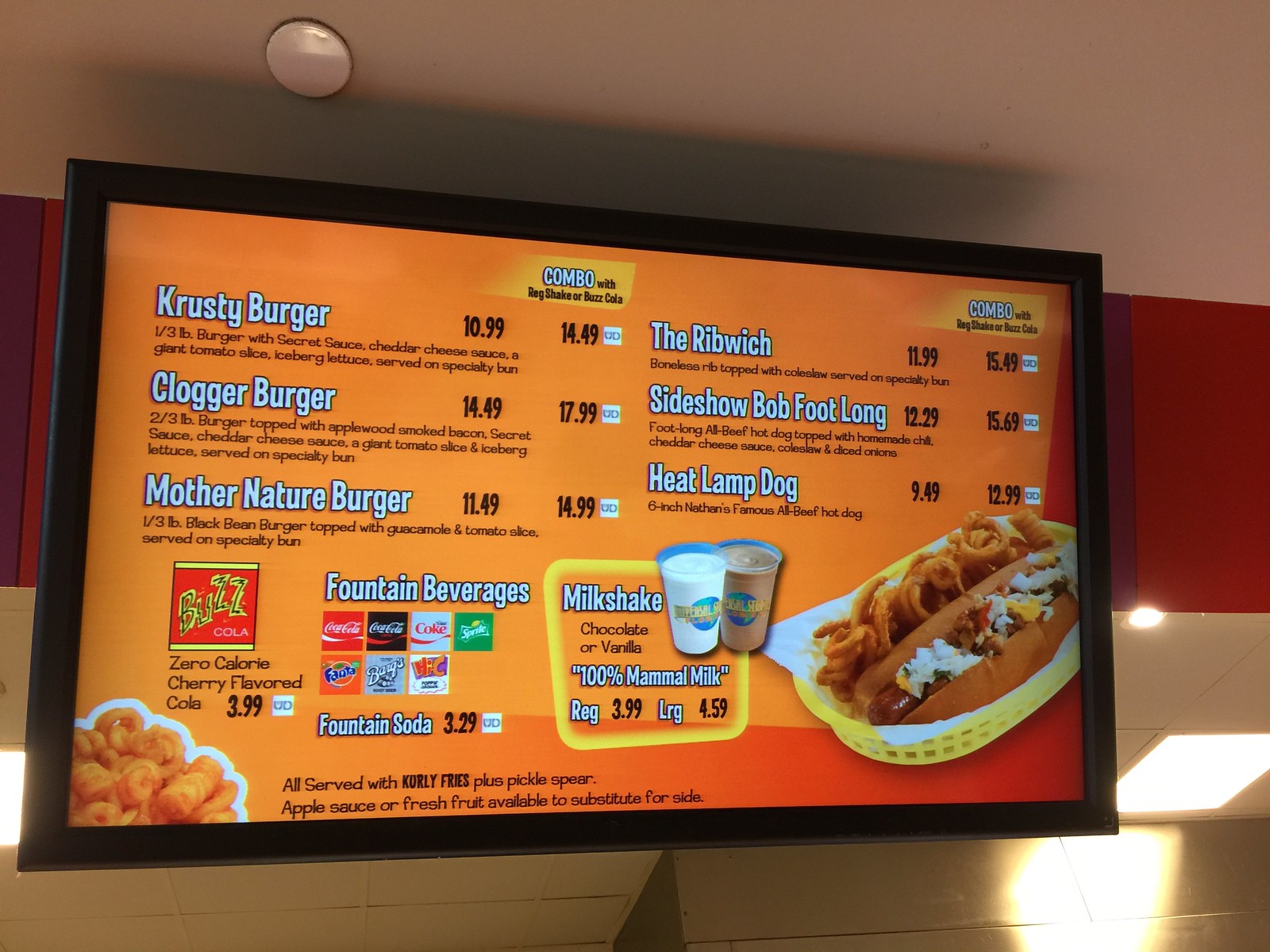The image depicts a detailed menu. At the top left corner, there’s a white circle. The background mostly displays a white tiled ceiling illuminated by a light shining down, casting a warm glow on the wall below. Prominently featured is a yellow rectangle with the word “Combo” written on it, suggesting combo meal options.

The first section of the menu reads:
- **Krusty Burger**: $10.99 or $15.49 for the combo
- **The Rib-Wich**: $11.99 or $15.49 for the combo
- **Quagga Burger**: $14.99 or $17.99 for the combo
- **Sideshow Bob Footlong**: $12.29 or $15.69 for the combo
- **Mother Nature Burger**: $11.49 or $14.99 for the combo
- **The Heat Lamp Dog**: $9.49 or $12.99 for the combo

On the bottom left of the menu, there’s a red square featuring “Buzz Cola” and below it, “Zero Calorie Cherry Flavored Soda.”

The right side of the menu lists fountain beverages:
- **Coca-Cola**
- **Coca-Cola Zero**
- **Diet Coca-Cola**
- **Sprite**
- **Fanta Orange**
- **Hi-C Orange**

These fountain sodas range in price from $3.00 to $3.29.

The menu also notes that all meals are served with curly fries and a pickle spear. There’s a section for sauces and other sides on the left which mentions curly fries. On the far right-hand side, there’s an illustration of a basket with a hot dog in it.

Additional menu items include:
- **Milkshake (Chocolate or Vanilla)**: $3.99 for a regular, $4.99 for a large

An image depicts two cups - one entirely white and the other all brown, likely representing the sizes or types of milkshakes available, emphasizing their use of 100% mammal milk.